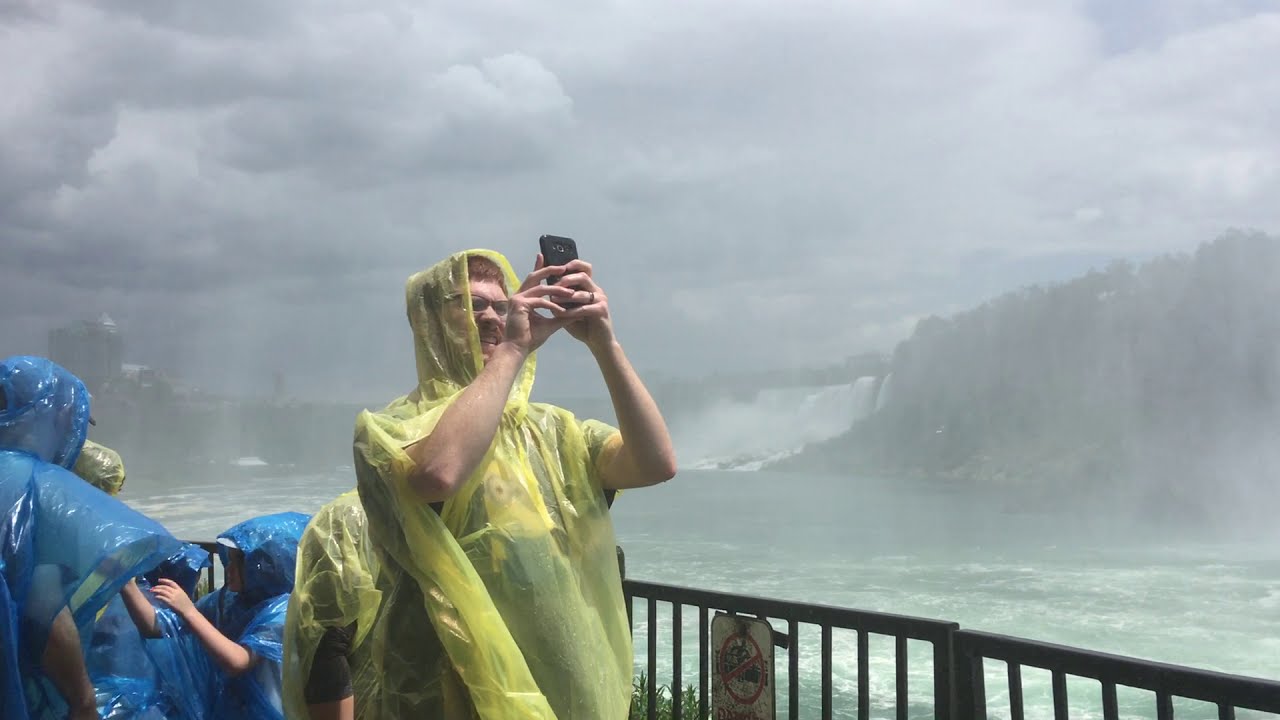In this detailed photograph, a group of four to five tourists, dressed in blue and yellow ponchos to protect themselves from the mist, are positioned in the bottom left of the image near a large waterfall. They have fair, peach-colored skin, and one individual on the far right is holding a black cell phone at face level, seemingly taking a photo or looking at something on the device. Behind them is a black metal guardrail with a small, mostly illegible sign that features some red, black, and white details, possibly prohibiting climbing. In the background, a vast body of turquoise water stretches out, with a prominent waterfall cascading down in white torrents. The scene is set under a dark, cloudy sky, creating a misty atmosphere that obscures some of the finer details, evoking a typical tourist site ambiance such as Niagara Falls.